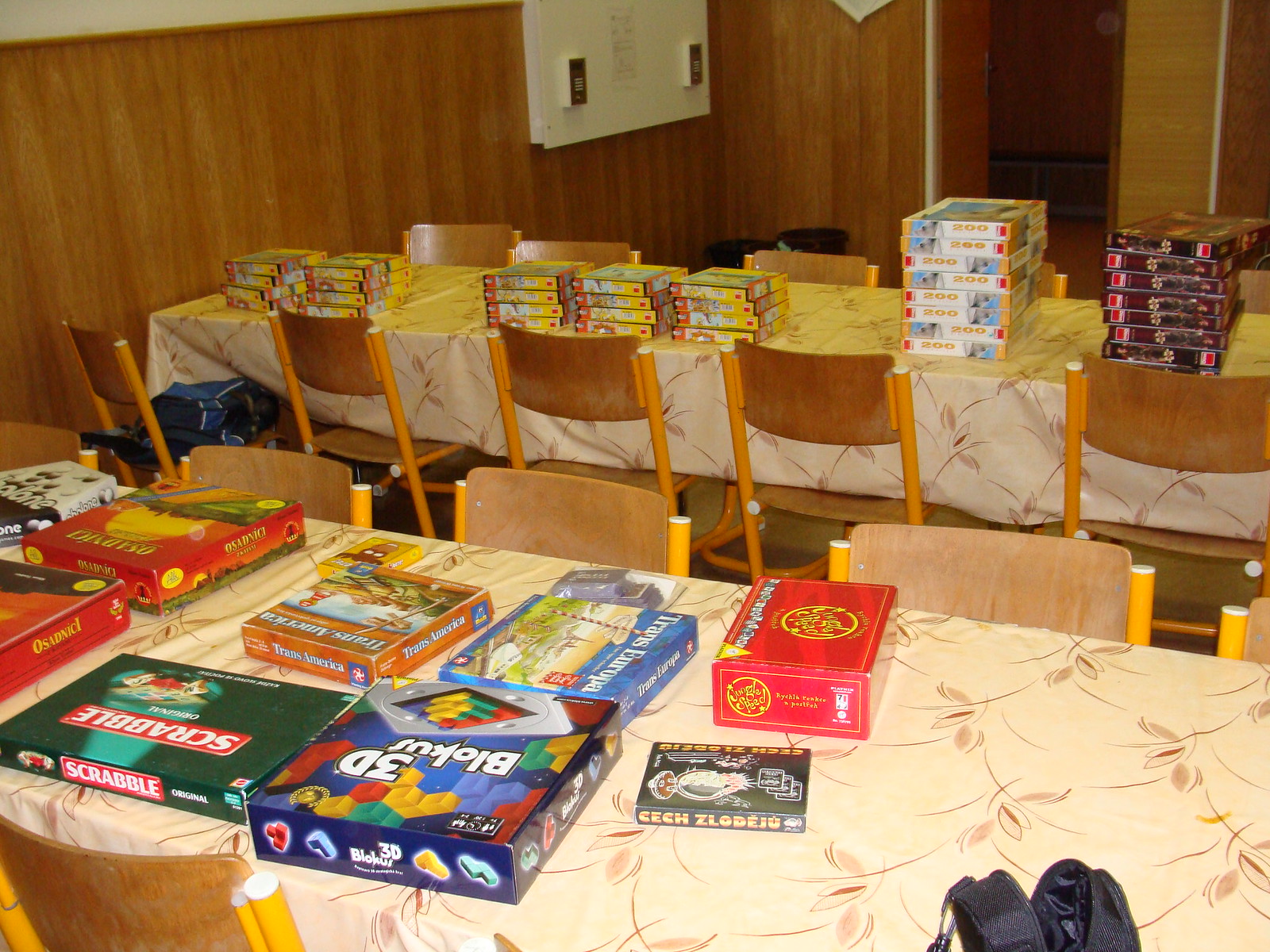The image showcases a likely cafeteria or library setting with two long tables extending beyond the frame. Each table is surrounded by wooden chairs with a total of at least eight visible. The tables are draped in beige tablecloths with patterned leaves and are cluttered with a mix of board games and puzzles. On the rear table, there are about 12 to 14 of one type of puzzle, four different puzzles lined up, and another stack of about eight. The forward table is more chaotic, with various board games such as 3D Block, Us, and Scrabble scattered across it. The room features wood paneling on the walls with a white object, possibly a circuit breaker, positioned on one side. A doorway is visible in the top right-hand corner, leading to another area, adding to the room's detailed, well-used ambiance.